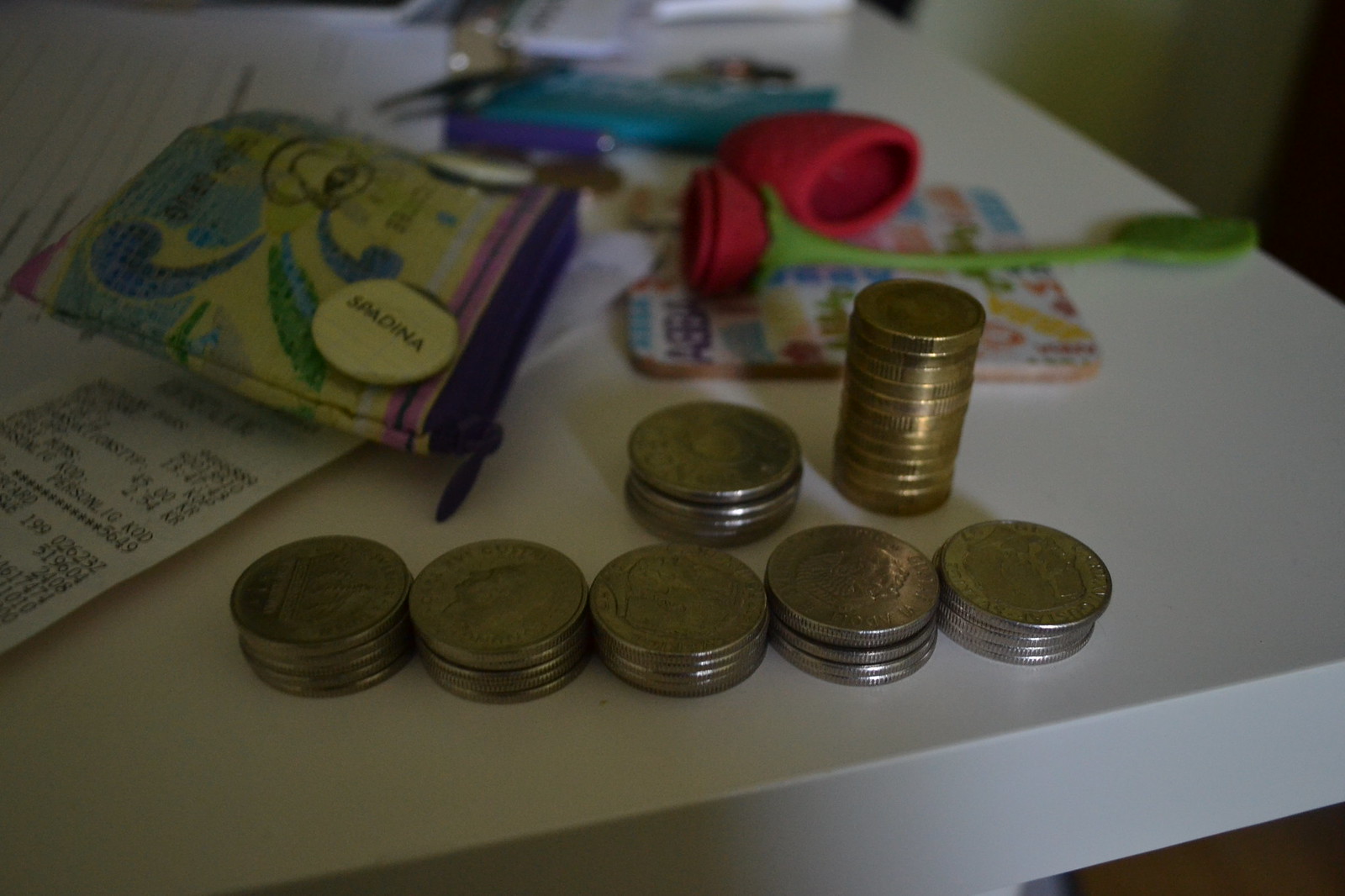In this photo, there is a close-up of the edge of a white plastic table cluttered with various objects that blend together in a blurry mess. The foreground is dominated by several stacks of coins, primarily quarters and dimes, with about seven distinct piles. There are also some nickel-sized gold coins arranged neatly in stacks. A small, colorful coin purse with a zipper, featuring purple, green, yellow, and blue hues, lies nearby. It is noted to have a little pin that says "Spadina" and a design including a flower, a cup of coffee, and possibly rubber roses. There are scattered papers and what appears to be a receipt, hinting at a recent transaction or purchase. A coaster with various words inscribed on it can also be seen among the clutter. The overall scene suggests someone has emptied their pockets and begun to count their coins, possibly after returning home.